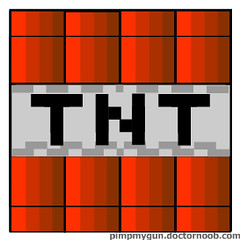This image appears to be inspired by the video game Minecraft, characterized by its pixelated and square-centric graphics. Centered within a square frame, the design prominently features four vertical red bands making a box-like structure, reminiscent of the items seen in classic platformer games like Mario. These bands are intersected by horizontal black lines both at the top and bottom, giving the appearance of a divided, compartmentalized object. In the center of this red and black structure is a large, gray label adorned with the text "TNT" in a bold, black font, stylized to fit a cartoonish or video game aesthetic. The background of the label contains a checkered pattern in varying shades of gray, enhancing the visual depth. The cross piece of the "T" in "TNT" appears broken into separated squares. At the bottom right corner of the image, there is a watermark that reads "PimpMyGun.DrNoob.com," indicating the source of the image. The overall structure and style strongly suggest a dynamite box, often associated with explosive in-game items, reinforcing its connection to Minecraft or similar video game genres.